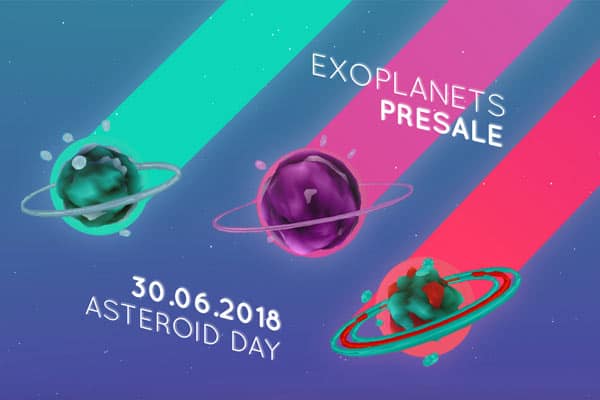The image is a poster with a gradient blue background, transitioning from a purple hue at the base to a teal blue at the top. In the bottom left corner, the date "30.06.2018" is displayed in white text, with "asteroid day" written beneath it. In the upper right corner, also in white text, is the phrase "exoplanets presale." From the top, three thick, bold lines descend diagonally across the poster. The top left line is light green, attached to a dark green planet with a silver ring. The middle line is pink, ending at a dark purple planet with a light purple ring. The rightmost line is red, extending close to the bottom of the image, leading to a green and red planet with a matching red and green ring.